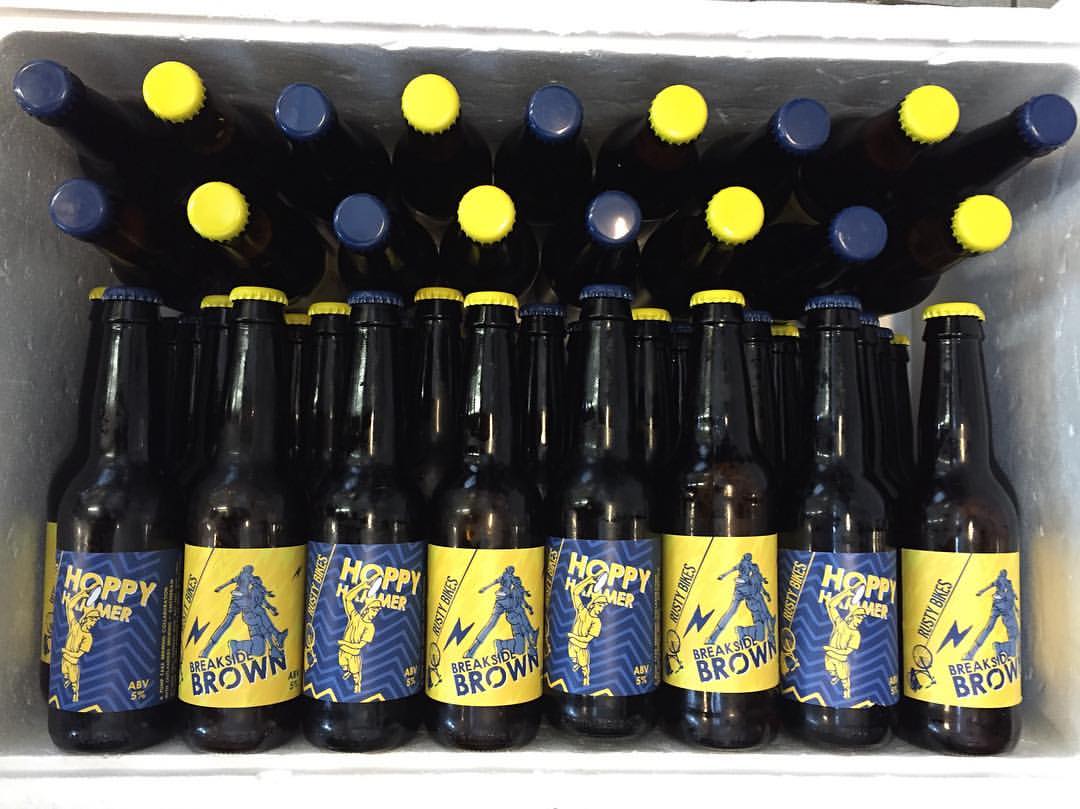This is a top-down view of the inside of a white styrofoam cooler filled with bottles of beer. The cooler is light in color with a white interior, and it has a slightly rugged texture with a few small chunks missing, suggesting it's a foam cooler. The bottles are neatly arranged in an alternating blue and yellow pattern. The bottles are aligned both horizontally and vertically, creating an attractive and organized display.

In the cooler, there are two distinct types of labels. The bottles with blue labels and blue caps have a design featuring zigzag chevron stripes and an illustration of a man in a dance pose with the label "Hoppy Palmer." The bottles with yellow labels and yellow caps depict two men in a martial arts stance with the label "Breakside Brown." The blue and yellow labels are muted and not overly bright, complementing each other well.

The horizontal arrangement on the bottom shows several rows of bottles lying on their sides, alternating blue and yellow. Above these, two rows of bottles are positioned vertically, displaying their blue and yellow caps. This arrangement enhances the visual appeal of the assortment, making it not only practical for cooler storage but also artistically pleasing.